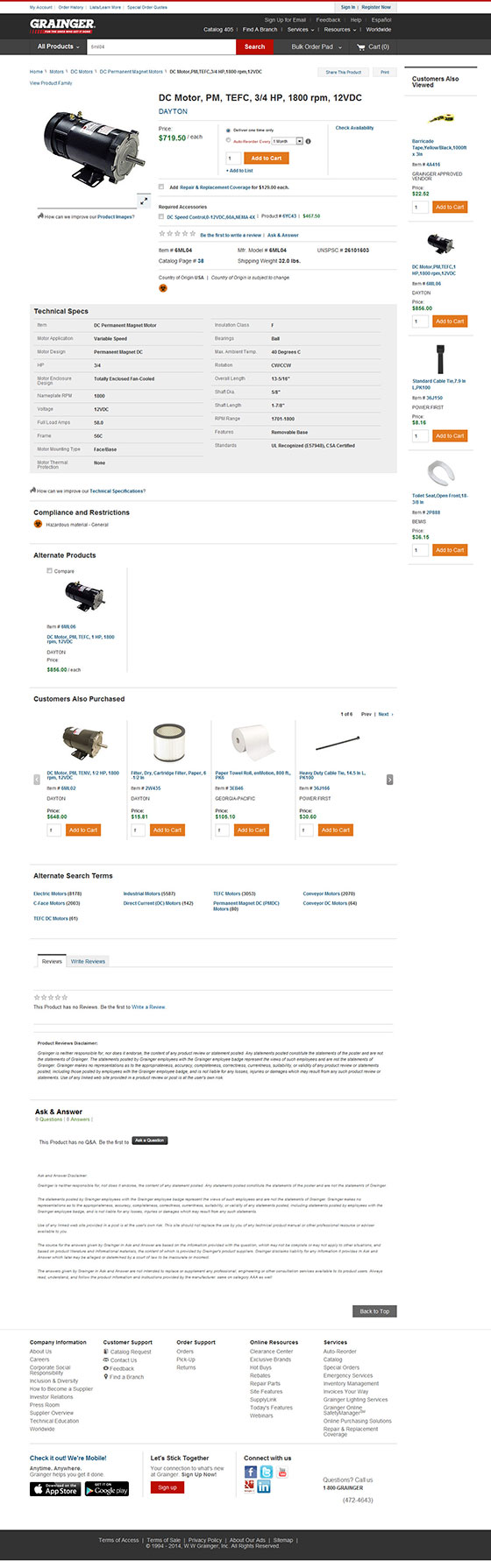This image depicts a stretched and low-resolution screenshot of the Grainger website, which severely impacts readability. The top of the page features a black navigation bar with the name "Grainger" displayed in white text. Numerous white links are present on this bar, leading to various sections such as "Find a Branch," "Services," "Resources," and "All Products." A white search bar with an adjacent red search button is also visible.

Below the navigation bar, there's a highlighted product listing for a "DC Motor, PM, TE, FC, 3/4 HP, 1800 RPM, 12 VDC, Dayton," priced at $719.50 each. The "Add to Cart" button is orange with white text, and there's an input box pre-filled with '1' to indicate the quantity.

Additionally, there's an option titled "Repair and Replace Coverage" priced at $129 each, accompanied by an "Add" button. The website layout includes other items and a specifications section, though the text is mostly unreadable due to poor resolution and distorted width.